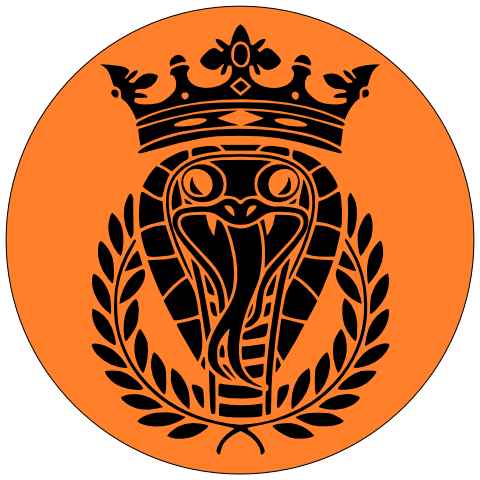The image is a digitally created logo, prominently featuring an orange circle with a thin black border on the outer edge, centered in a white space, giving it a floating appearance. Within this circle, a stylized cartoon black cobra head is depicted, positioned centrally. The cobra, visible from its upper neck to the top of its head, has menacing eyes and an open mouth from which a long forked tongue extends down its body. Beneath the cobra head are two semi-circular black wreaths, adding a touch of regality to the design. Above the cobra, a detailed black outline of a crown hovers, adorned with three diamond shapes on the center band and multiple pointed spikes at the top. The entire image uses a limited color palette of black and orange, contributing to the bold, striking appearance of the logo, suitable for a company brand, flag, or even a cryptocurrency icon. The minimalist yet impactful design is void of any text, ensuring the image's elements—crown, snake, and wreaths—are the focal points.